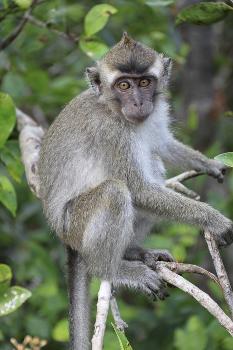In this vertically aligned, photorealistic photograph taken in the wild, a small, engaging monkey is perched in a tree surrounded by abundant greenery. The monkey, characterized by its gray fur and white patches around the temples, chest, and stomach, is squatting on a forked branch. Its head is adorned with small, visible ears and a distinctive spike of hair, giving its facial features a very engaging appearance. The monkey's muted yellow eyes and elongated face create an expressive look as it gazes directly at the camera, despite its body facing the right side of the image. Its long, shaggy tail hangs down beneath it, while its front hands and a back foot grip the light-colored branch for support. In the background, out-of-focus leaves add to the natural setting, emphasizing the lush, green environment. The photograph, taken during the afternoon, captures the essence of this small monkey's demeanor as it seemingly poses for the camera amidst its leafy habitat.